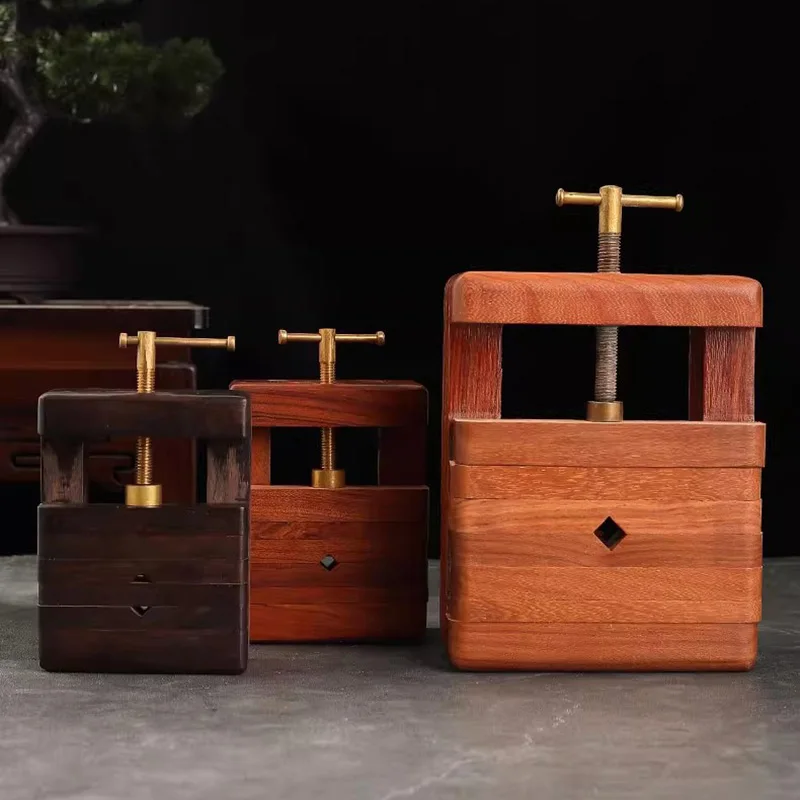This photograph, taken indoors, features a serene and detailed setting. The square image, approximately six inches by six inches, is partially blacked out at the top. On the left side of the image, a dark cherry wood table or stand is visible, supporting a small bonsai plant housed in a very dark brown or black pot. Below this, a stone gray table with light gray striping and cracks commands the lower portion of the frame.

On this gray table, three wooden vices are meticulously arranged. Each vice is rectangular and features a metal rod at its center, which is capped with a crossbar rod used to spin and press the wooden pieces together. The vice on the far left is the smallest, crafted from dark mahogany wood. The center vice, resembling the size of the first but appearing slightly elevated due to its placement, is made from redwood. The rightmost vice is the tallest and fashioned from medium brown wood. These vices are designed to securely hold small objects or pieces of wood in place while they are being worked on, featuring screws that, when turned, separate the wood sides to accommodate various shapes and sizes of workpieces.